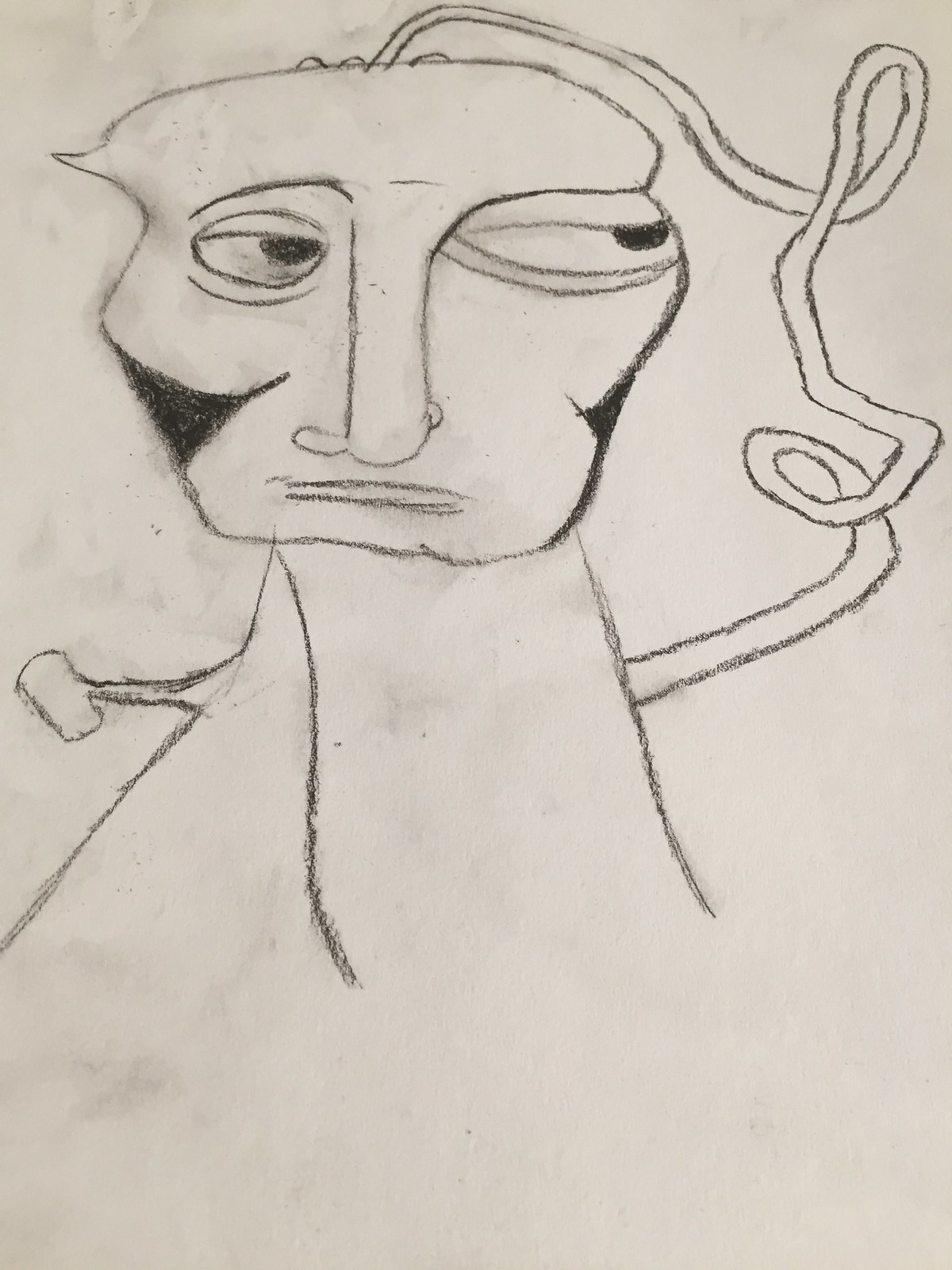The image is a surrealist pencil or charcoal drawing on an off-white canvas, with some smudges visible. The artwork features an abstract, misshapen face with asymmetrical eyes; the right eye is elongated and twice as large as the left, both glancing to the right. The face has darkly shaded cheekbones, an unevenly long vertical nose, and a simple two-line mouth. The head appears pointed on the left side, with some squiggly lines on top, possibly representing hair. From the neck, a crude hand extends, holding a cup, while the left arm twists and loops upward, ending with a hand scratching the head. The overall composition creates a slightly unsettling, stylized appearance.